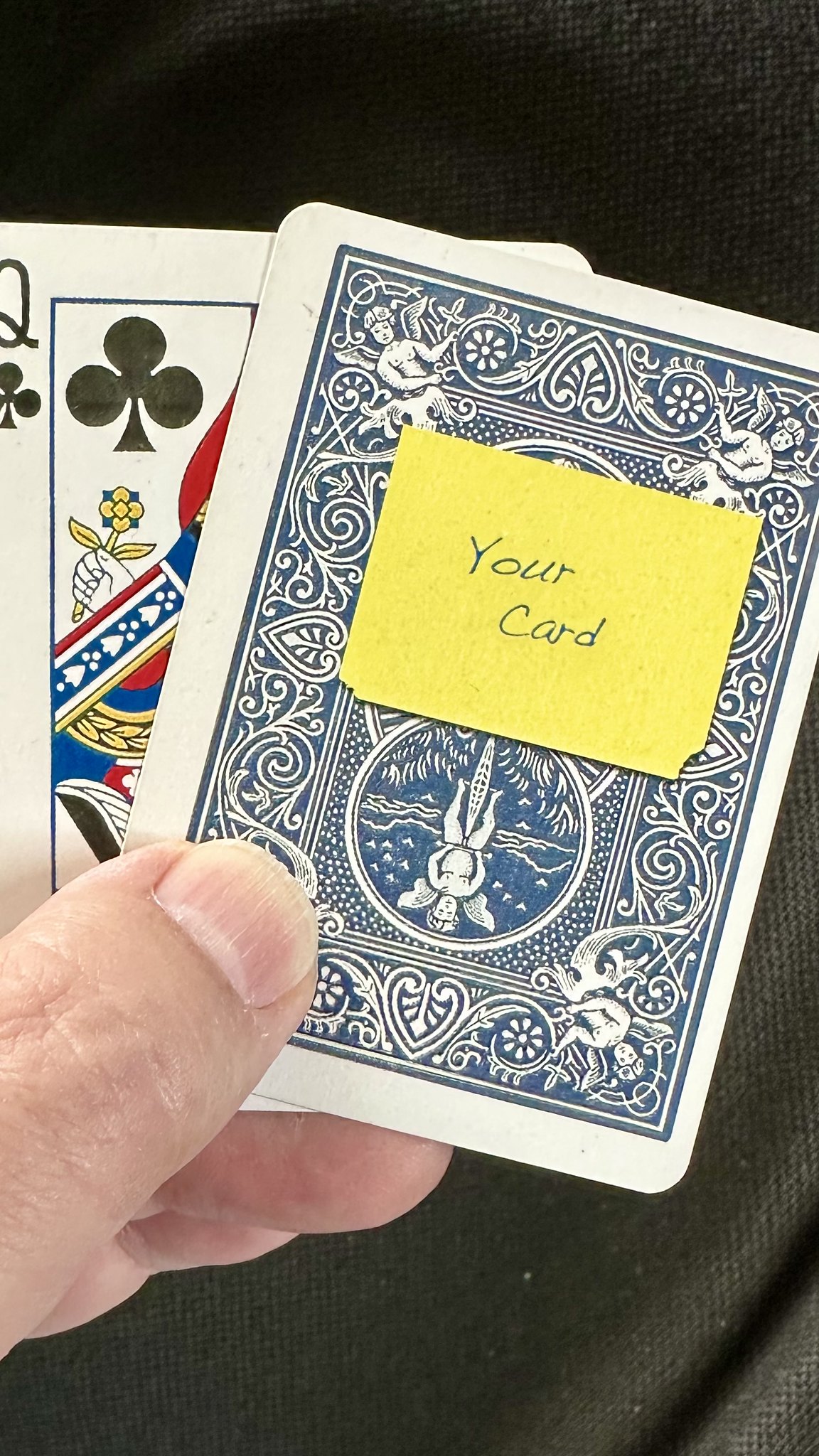The image depicts a person holding two playing cards in their left hand. The hand is positioned to reveal the thumb and the tips of the pinky and ring fingers curling around the cards. The thumb is bent over, firmly grasping the cards which are visible in part. 

The bottom card is a Queen of Clubs, identifiable by the partial display of the letter 'Q' and the club symbol on a black background. Only the left side and the upper right corner of this card are visible. 

The top card, which partially obscures the Queen of Clubs, has a distinctive design featuring a white border encircling a blue field adorned with intricate white swirls and heart patterns. A thin white line separates a larger blue border from the decorative central part of the card. This top card also has a small, yellow sticky note affixed to it, with the handwritten message "Your Card," where both the 'Y' and 'C' are capitalized.

The entire scene is set against a stark black background, emphasizing the details of the cards and the hand holding them.